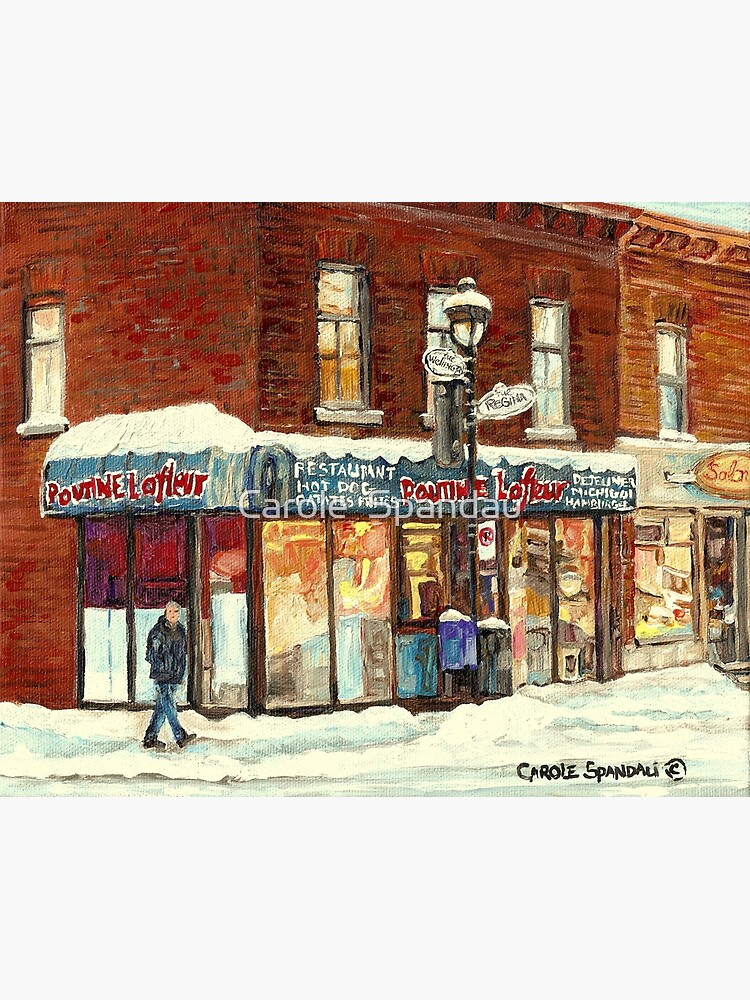This artwork, possibly a print or painting, depicts a quaint town square blanketed in snow. Central to the scene are two red brick, two-story buildings with retail stores on the ground floor and potential residences above. Prominent among the establishments is a restaurant with a green awning bearing the words "restaurants," "Poutine," "La Fleur," and "hot dogs" in large light-colored letters. On the corner, a classic black street lamp with a white glass globe illuminates the area, while oval street signs mark the intersection. The storefront windows glow warmly, casting orange, red, and white hues. A solitary figure dressed in a black or navy parka, jeans, and boots, with blonde hair, walks through the snow past the buildings. Next to the restaurant, possibly a hardware store or salon, adds to the old-town charm. The bottom of the image is signed by the artist, "Harold Spandale," alongside a copyright symbol.